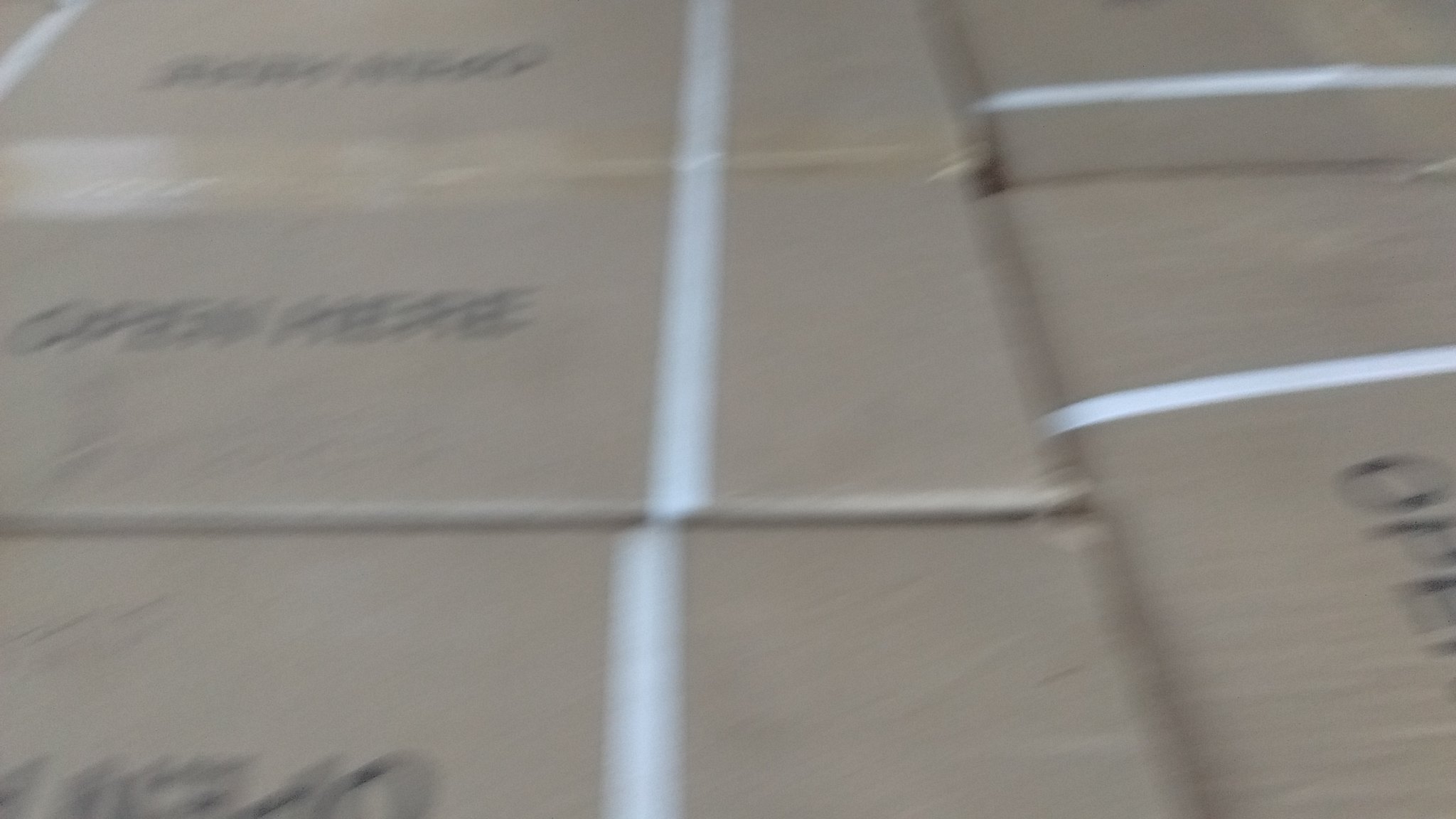The image features a grayish background with a set of rectangular objects arranged in a specific pattern. On the left side, these rectangular items are stacked horizontally, while on the right, they appear to be stacked vertically. Running through these objects are white and light bluish lines that resemble plastic straps. A noticeable gap is present between two of the boxes in the upper right corner, revealing a black area in the void between them, indicating they are not tightly packed. In the center of these rectangular objects, there is some black lettering that is indistinct due to blurriness, though an "O" and what appears to be a "P" can be discerned, along with possibly some numbers.